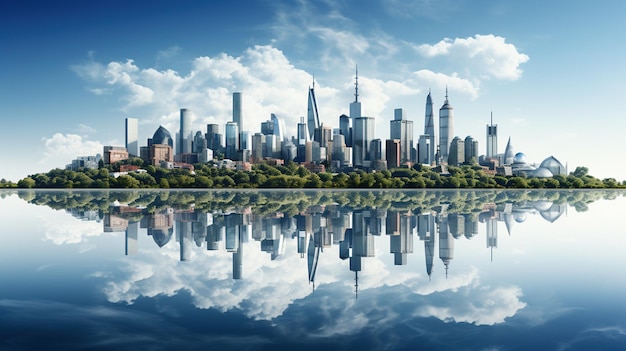The image depicts a digitally rendered, futuristic cityscape situated on an island. This city features a striking array of tall skyscrapers and futuristic buildings of various shapes, including sleek, slanted structures and cylindrical forms, many with antennas stretching towards the sky. The island itself is encircled by lush greenery, accentuating the advanced urban center located at its heart. The surrounding water, with its deep blue hues, mirrors the entire cityscape and the blue sky above, creating a seamless reflection that makes it difficult to discern the upright orientation. Billowing white clouds adorn the sky, adding to the serene yet advanced atmosphere of this visionary landscape.